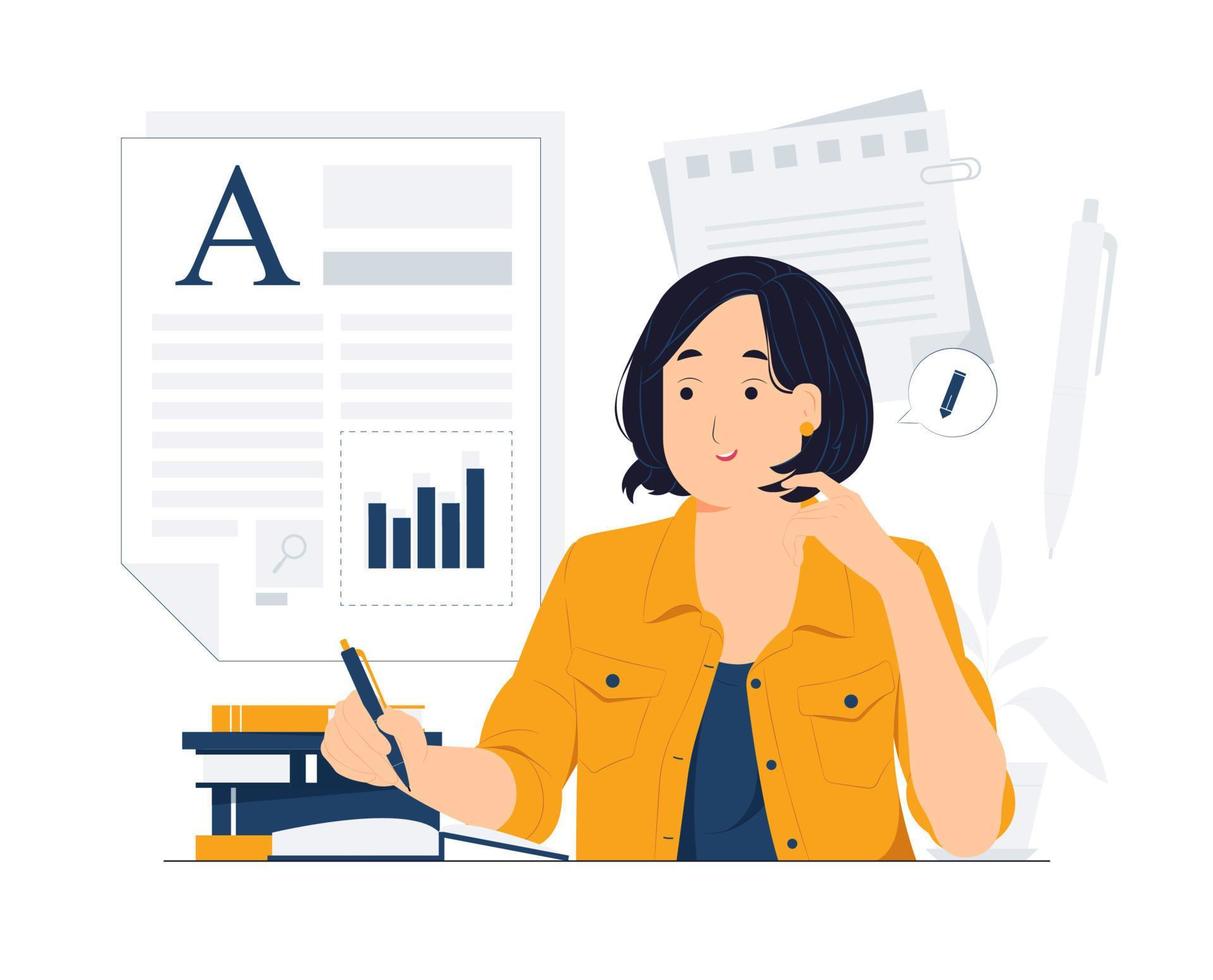This detailed cartoon illustration depicts a woman with short, dark hair that falls to her chin. She is seated at a desk, facing left and looking slightly down. She wears an open yellow jacket with blue buttons over a dark blue blouse, with the sleeves of the jacket pulled up to just below her elbows. Her right hand holds a pen, poised above a blue-covered book in which she appears to be writing. Surrounding her are various other books, some with blue covers and others with yellow covers. 

A speech bubble emerges from her, containing an illustration of a pencil or pen, emphasizing her writing activity. Behind her, faint images of various gray papers are visible. One prominent paper extends from the center left of the picture up to the top, featuring a large letter 'A', blue text at the top, and a bar graph in the lower right corner. Additionally, there is an orange earring visible as her head is slightly turned. 

In the upper left corner, a book rests on a small stand. Also visible, superimposed behind her head, is a notepad held together by a paper clip. The light, shadowy image of a pen can be seen in the far right. Her left hand is up to her face, suggesting she is in deep thought or contemplation. The composition conveys a studious and reflective atmosphere, rich with scholarly elements and details.